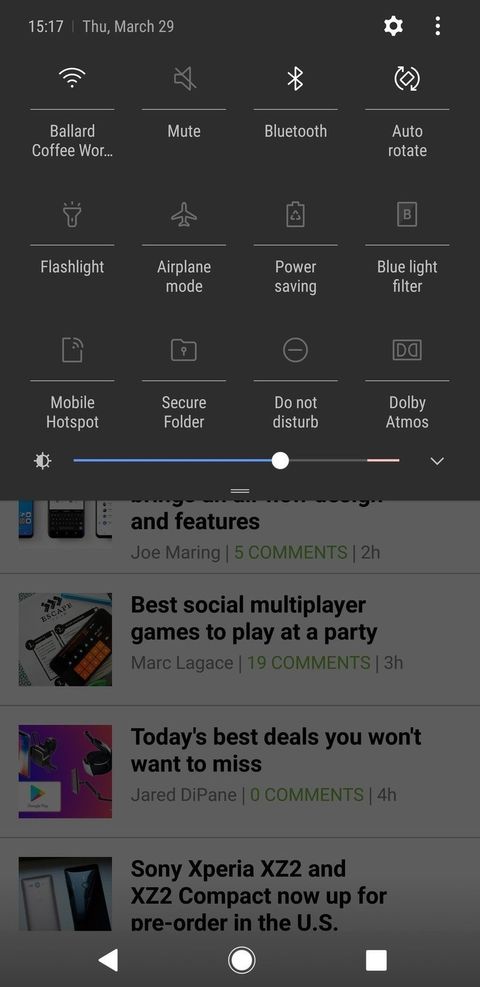The image depicts a cell phone screen with the top notification bar pulled down, revealing various controls and information. The time displayed is 15:17 on Thursday, March 29th. Just below the black notification bar, several control icons are visible, including Wi-Fi, Bluetooth, Auto Rotate, Flashlight, Airplane Mode, Power Saving, Blue Light Filter, Mobile Hotspot, Secure Folder, Do Not Disturb, and Dolby Atmos. The brightness level is set to approximately three-quarters, indicated by a blue progress bar, with the higher end marked in light red, signaling increased battery consumption. Below the notification controls, content suggestions are listed, including "Best Social Multiplayer Games to Play at a Party," "Today's Best Deals You Won't Want to Miss," and information about "Sony Xperia XZ2 and XZ2 Compact, now up for pre-order in the U.S."